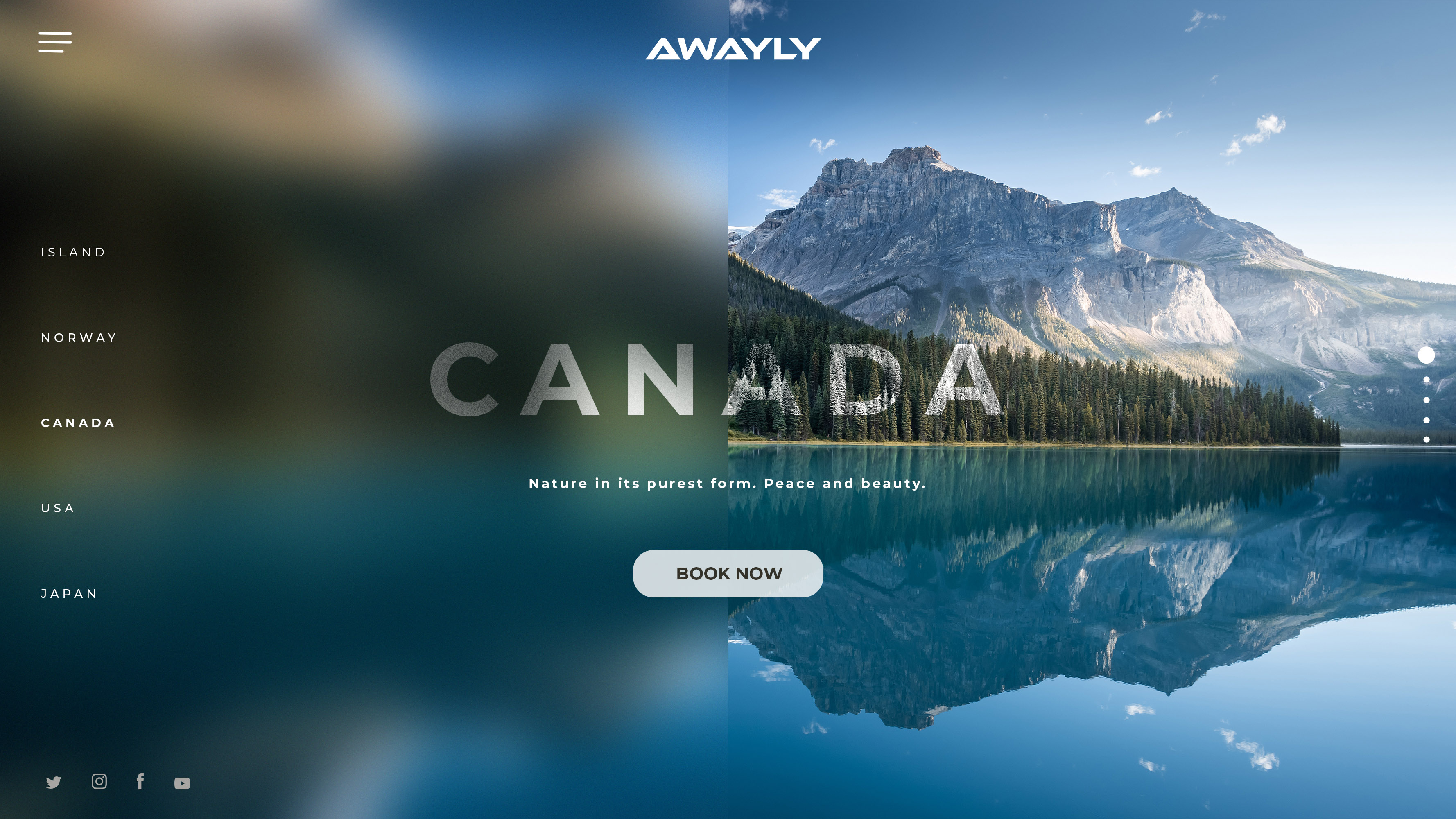Homepage of Awayly (A-W-A-Y-L-Y) Travel Website

The captivating homepage of the Awayly travel website presents a striking combination of clear and blurred elements, creating a visually engaging effect. At the top left corner, a hamburger menu provides easy navigation. Below it, a vertical list of destinations reads: Island, Norway, Canada, USA, and Japan, offering a glimpse into the travel options available.

Dominating the center of the image is a breathtaking snow-capped mountain range, bordered by verdant, tree-lined foothills. The word "Canada" is prominently displayed across the mountains, underlining the highlighted destination. Beneath this, the tagline "Nature in its purest form—peace and beauty" invites users to explore further.

At the foot of these majestic mountains lies a serene lake, so calm it mirrors the peaks like glass. The backdrop of a clear sky, with only a few wispy clouds, enhances the tranquility of the scene. A prominent "Book Now" button entices visitors to plan their adventure.

At the bottom of the page, icons for Twitter, Instagram, Facebook, and YouTube connect to Awayly's social media profiles.

Overall, this visually stimulating and descriptive layout underscores Awayly's focus on nature-driven travel experiences, with Canada as the featured destination among a range of global travel options.